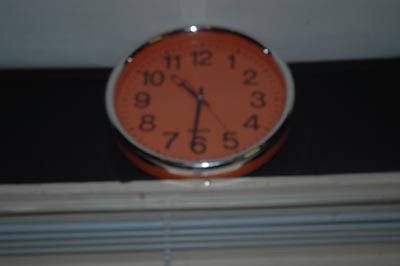The image displays an old-looking analog clock prominently positioned on a white shelf that appears to be at a significant height. The clock features a near-silver perimeter and a distinctly orange face with black numbers and hands, indicating the time as 10:31. The clock's background includes a dark green or black wall, and it is mounted above a window with visible blinds. The roof in the background is white. The overall scene is accented by various reflective coatings on the clock itself and the presence of four white tubes running horizontally beneath the shelf. There is also some unreadable text at the bottom of the clock's face.